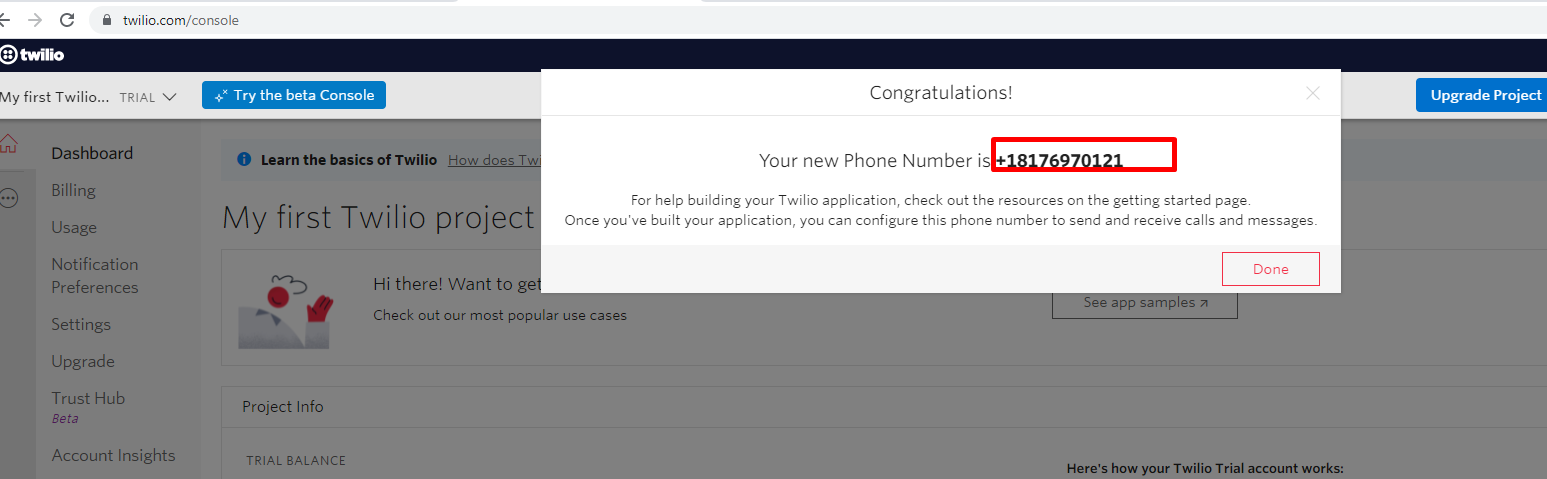This image is a highly detailed and descriptive screenshot of a desktop web browser window displaying the Twilio console. At the top left corner of the browser interface, there are navigation arrows: a darker, partially visible left arrow, and a light gray right arrow. Adjacent to these is a circular reload symbol. The browser's address bar, with a light gray background, displays the URL "twilio.com/console" alongside a dark gray lock icon, indicating a secure connection.

The upper section of the webpage features a thin, dark-colored bar—possibly navy or black—where "Twilio" is written in white font along with the brand's distinctive circular logo containing four shapes. Below this is a light gray bar with dark gray text that reads "my first Twilio..." followed by "trial" in a lighter gray font and a downward-pointing arrow, suggesting a dropdown menu. Within this section, there are two blue boxes: one on the left side encouraging users to "try the beta console," and another on the right prompting users to "upgrade project."

Partially obscuring this bar and extending into the area below it is a prominent white box displaying celebratory text: "Congratulations!" followed by an exclamation point, signaling a notable message or milestone within the user’s Twilio account.

Overall, this image encapsulates the user interface of the Twilio console, featuring navigational elements, brand-specific design components, and user account information, all presented in a structured and visually distinct layout.